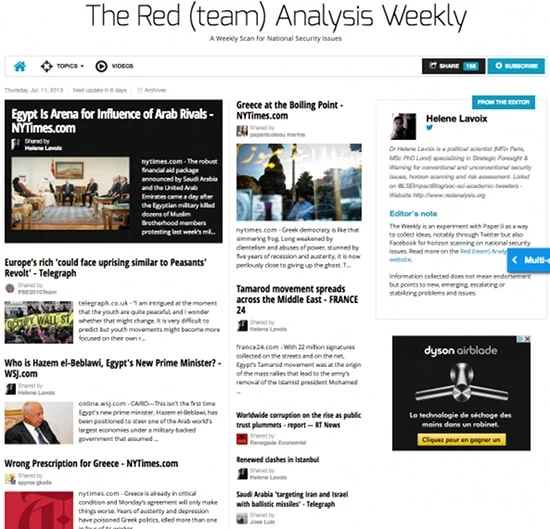This image is a detailed screenshot of a website that resembles a news aggregation platform. At the top of the page, prominently displayed in bold black letters is the title "The Red (Team) Analysis Weekly." 

In the upper left corner of the page, there is a prominent article set against a black background with white text. The headline reads: "Egypt is Arena for Influence of Arab Rivals," sourced from newyorktimes.com. Accompanying this article is a thumbnail picture depicting a formal room with several men in suits seated on chairs and sofas, engaged in conversation.

Other articles populate the page, displayed with black text on white backgrounds. Many of these articles are sourced from the New York Times, although there are contributions from other newspapers as well. One notable article features the image of an older white man in a suit alongside the headline: "Who is Hazim El-Bawal, Egypt's New Prime Minister," attributed to WSJ.com. Below this, there is additional text in black.

The layout of the page is organized into three columns, each containing a mix of articles, some with accompanying images and others without.